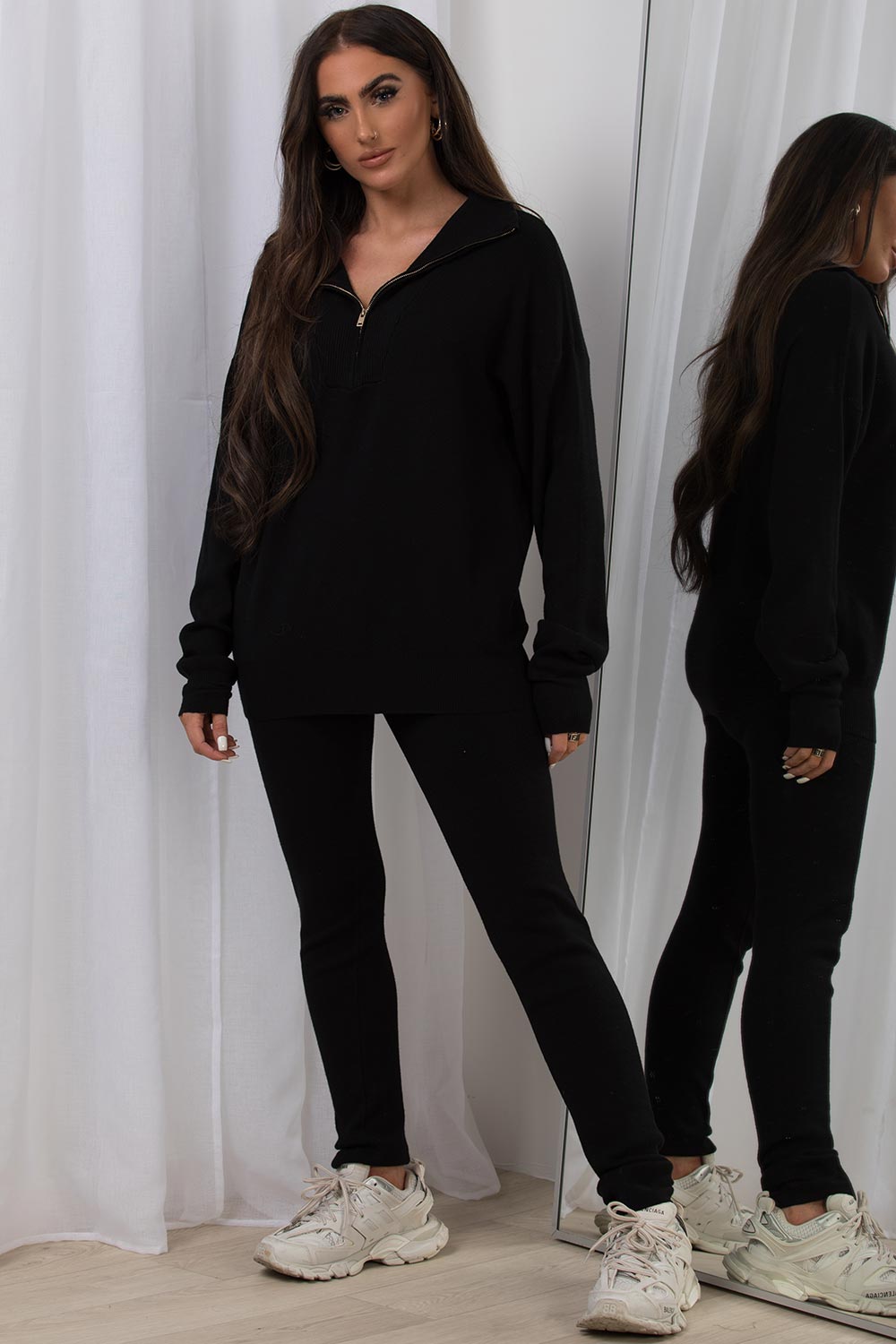The image features a woman standing in what appears to be a dressing room. She is positioned in front of a white, slightly sheer drape on her left and a floor-length mirror leaned against the wall on her right, reflecting her back and side. She is wearing a black tracksuit consisting of a zippered long-sleeve sweater, which is slightly unzipped in a V-neck style, and black leggings or tight-fitting pants. Her attire is complemented by white jogging shoes. The woman, who has dark brown hair and thick eyebrows, appears tanned with a neutral, serious expression on her face. She has a nose piercing, earrings, and is adorned with white nail polish and a ring on her middle finger. The floor beneath her appears to be tiled, reinforcing the dressing room setting.